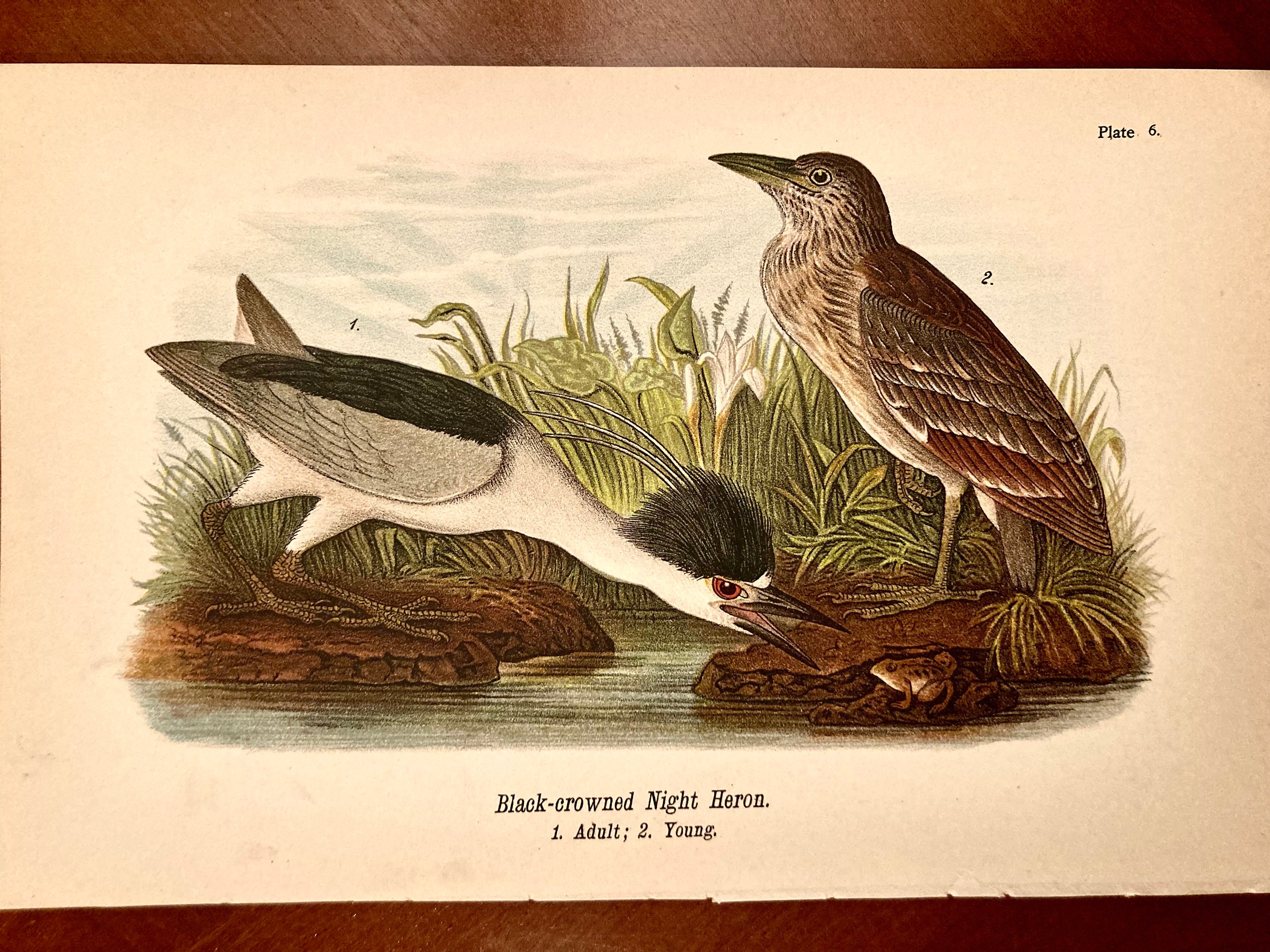The image is a detailed vintage drawing of a marshy grassland scene labeled "Plate 6.” It features a pair of black-crowned night herons standing by some rocks near a stream or pond, surrounded by lush vegetation. The background is bordered by brown strips at the top and bottom, with a very light beige or peach hue filling the center.

The central focus is on two birds: an adult black-crowned night heron and a young one. The adult heron is facing right, distinguished by its sharp pointed beak aimed at a small frog on the ground, suggesting an impending meal. It showcases striking features including a long neck, black and gray wings, black feathers sticking up from its head, and three long decorative feathers extending from its crown. The young heron, standing to the left and facing in that direction, has its wings down and is predominantly brown with a smooth head and a less pronounced beak. The text beneath the birds reads, "Black-crowned night heron, one adult, two young," indicating the age difference and labeling the species. The upper right-hand corner of the page is marked "Plate 6."